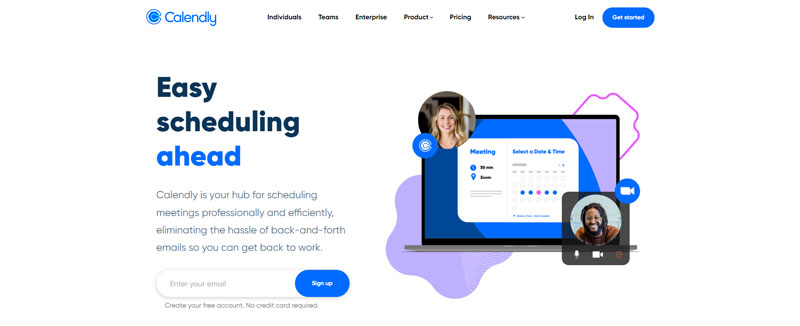The upper left portion of the webpage features the main navigation menu, which includes the following options: "Calendly," "Individuals," "Teams," "Enterprise," "Product," "Pricing," "Resources," "Login," and a prominent blue "Get Started" button. 

On the left side of the page, a bold headline reads "Easy Scheduling Ahead." Below this, a description explains that "Calendly is your hub for scheduling meetings professionally and efficiently, eliminating the hassle of back-and-forth emails so you can get back to work." An "Enter Your Email" field is available for users to sign up, accompanied by a blue "Create Your Free Account" button, with a note indicating that no credit card is required.

In the lower right corner of the image, there's a picture of a girl with blonde hair and a guy with dreadlocks. Within the computer screen in the image, a scheduling interface is displayed, with the words "Meeting, Select a Date and Time," and a visible calendar for selecting a date and time.

This comprehensive view meshes together both the user-friendly design and the personable touch of Calendly's interface, captured clearly in the image.